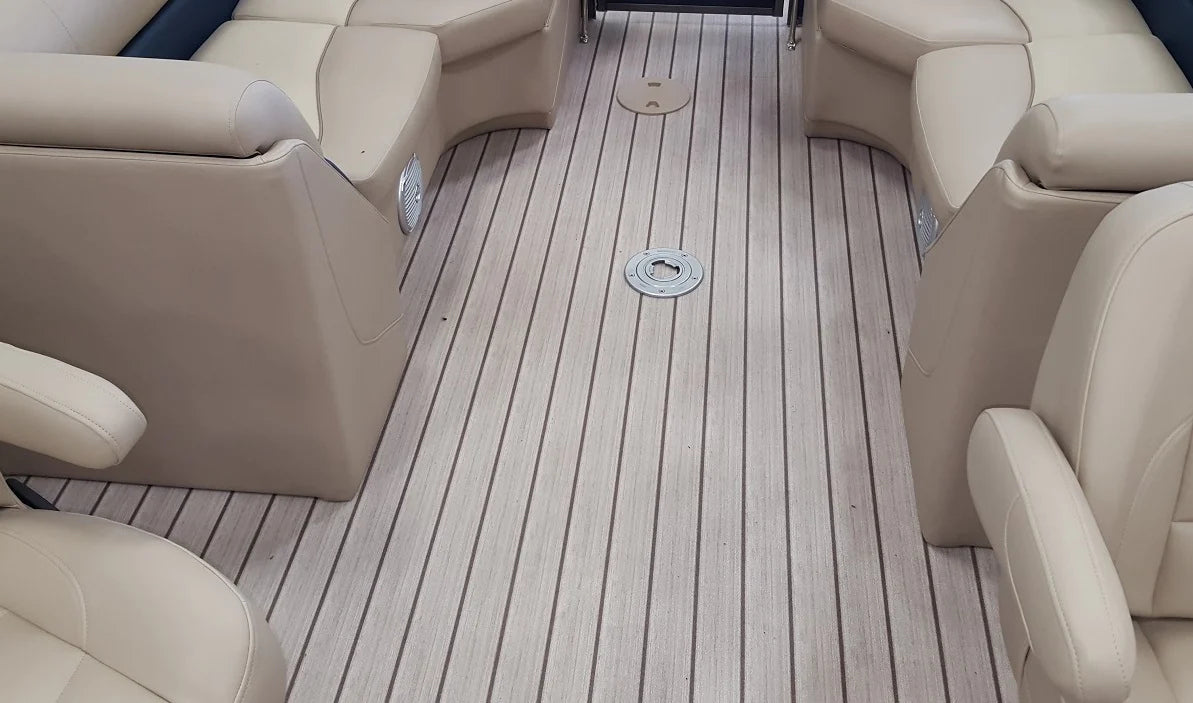The image depicts the deck of a boat, centered around a faux wood floor with vertical, dark stripes running up and down. In the upper left and upper right corners, there are cushioned bench-style seats upholstered in a light beige material. Additionally, matching beige-colored cushioned chairs with movable armrests are located in the bottom left and bottom right corners. Notably, the floor features cleats, which are integral to boats, with one cleat plate made of stainless steel and another of brass. The detailed teak-like flooring and the arrangement of seating create a unified and practical design characteristic of a vessel's interior space.